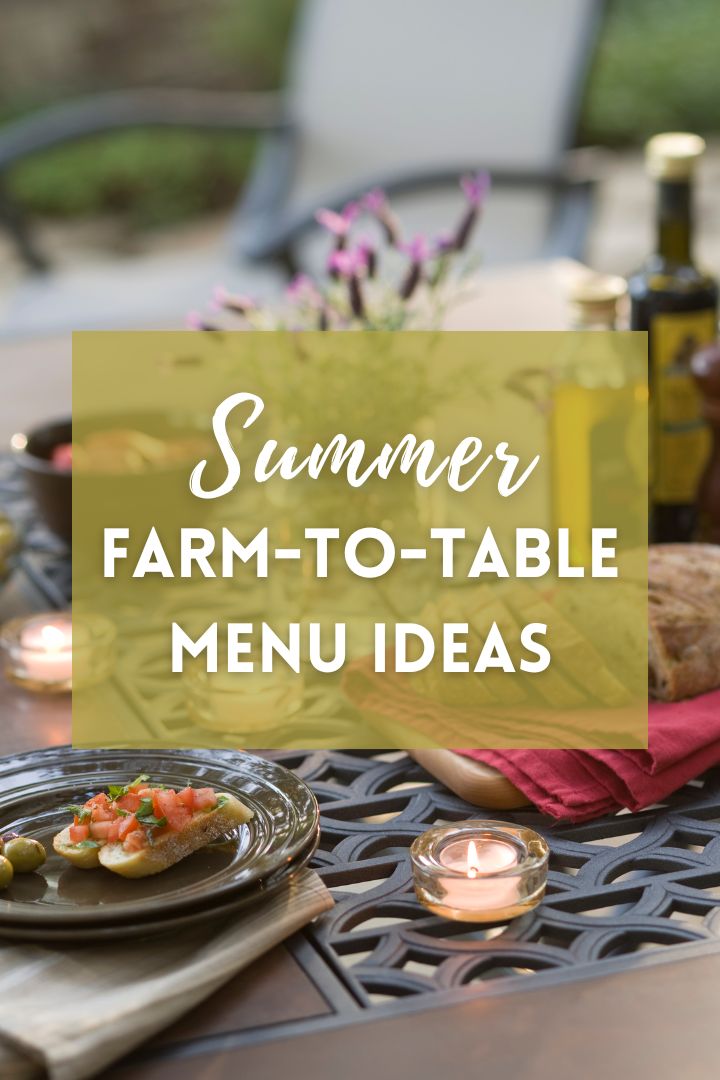The image is a beautifully arranged outdoor tablescape, primarily designed as a social media graphic for a blog or an advertisement. The foreground features a well-lit table with two green plates stacked on a white folded napkin, adorned with bruschetta and two green olives. Tea light candles on clear holders, three in total, are placed on the table, though only one is in sharp focus. A block of transparent yellow with white lettering prominently displays the text "Summer Farm-to-Table Menu Ideas."

The midground showcases a French-looking tabletop with brown tiles and an assortment of tableware, including a bowl and a plate of food. Laying on a folded red napkin on a brown cutting board is sliced French bread. Additionally, oil and vinegar bottles can be seen, and purple lavender flowers add a touch of greenery.

The background, intentionally blurred to draw focus to the table, hints at a chair and greenery surrounding the scene. The overall ambiance suggests a charming, rustic outdoor setting perfect for a summer meal. The image blends clarity and artful blur to emphasize the inviting table setup.